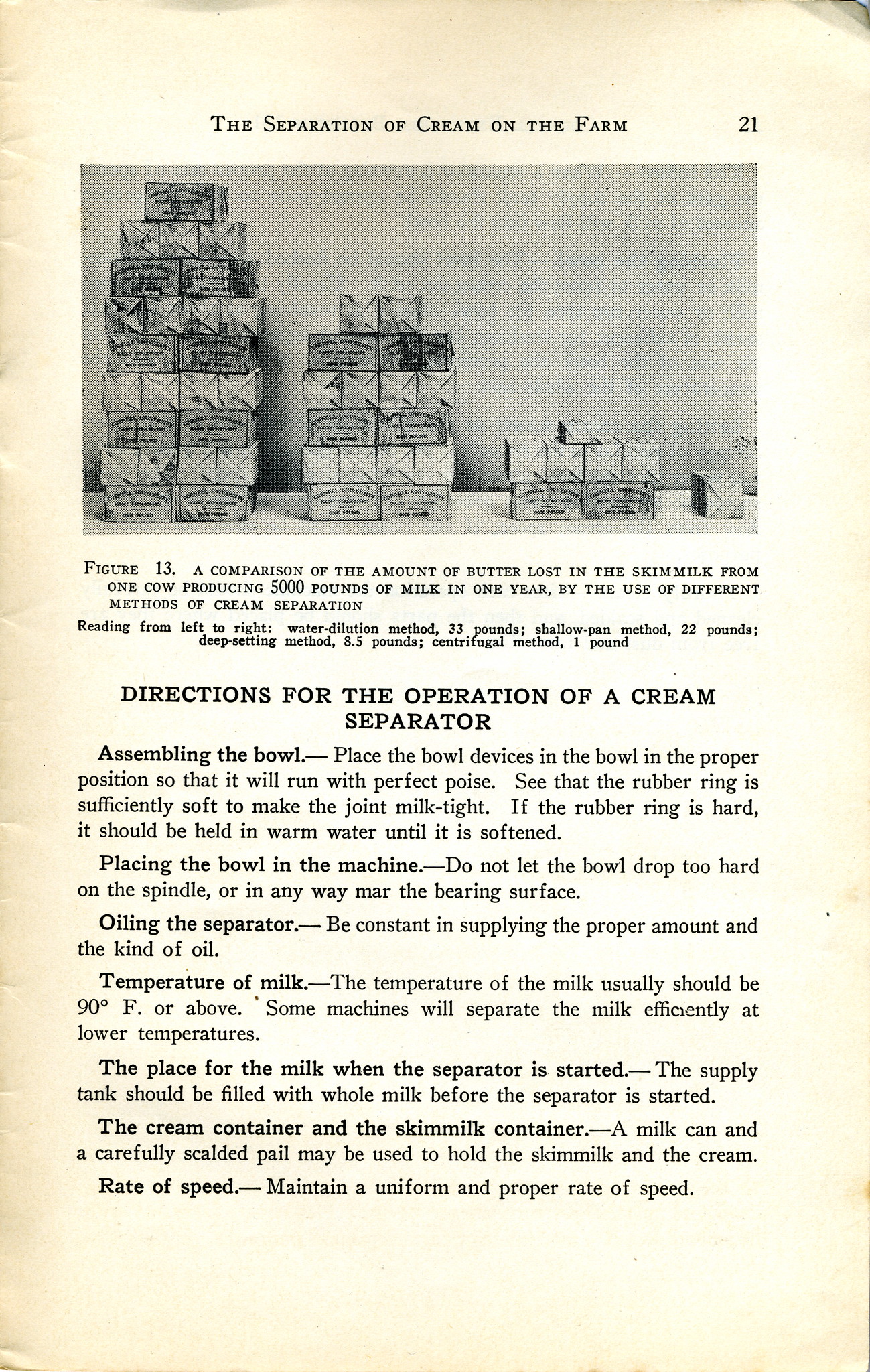This is a photograph of an aged, yellowed page from a book, identified as page 21 in the top right corner. The page features a heading at the top titled "The Separation of Cream on the Farm." Below the heading, there is a black-and-white photograph labeled "Figure 13" that appears to show various stacks of boxes. These boxes visually represent a comparison of the amount of butter lost in the skim milk from one cow producing 5,000 pounds of milk in a year using different methods of cream separation, with taller stacks indicating greater losses.

The detailed caption under the photograph explains the different methods and their respective butter losses: the water dilution method loses 33 pounds, the shallow pan method loses 22 pounds, the deep settling method loses 8.5 pounds, and the centrifugal method loses just 1 pound.

Further down, the page is titled "Directions for the Operation of a Cream Separator," providing meticulous instructions. It details the assembly of the bowl, ensures the rubber ring is soft and milk-tight, and warns against damaging the bowl during placement. The instructions also emphasize proper oiling of the separator, maintaining the milk temperature ideally at 90 degrees Fahrenheit, and filling the supply tank with whole milk before starting the machine. Additionally, it covers the proper handling of cream and skim milk containers, ensuring they are clean and maintained at a consistent operational speed.